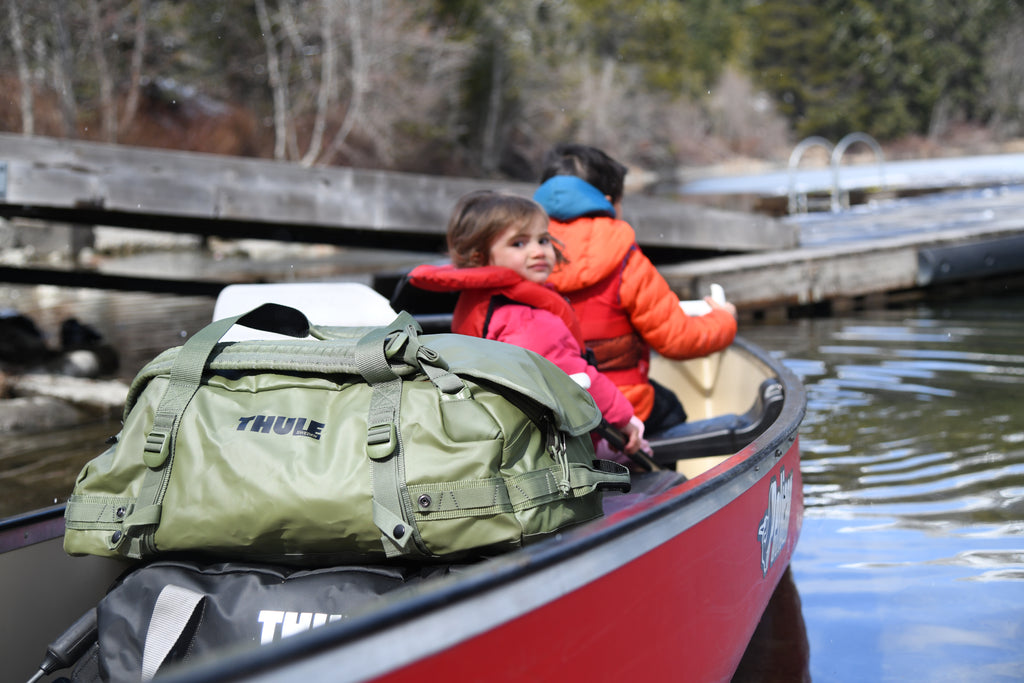In this color photograph, we see two individuals in a red canoe floating on calm waters, possibly on a lake. The water shows gentle ripples, adding to the serene setting. The surrounding background features a mix of lush green trees and some dried, grayish plants, adding texture to the scene.

The canoe is occupied by a little girl and an older person. The little girl, positioned towards the rear, has brown hair and wears a pink jacket along with a small red life jacket, adding a touch of vibrancy to her appearance. She is gazing backward at the camera, her curious expression captured in the moment. In front of her, facing away, is another person whose identity is more ambiguous; they have short black hair and are dressed in an orange winter coat. A blue hood from an underlying sweatshirt peeks out from beneath the coat, adding contrast.

A significant feature in the canoe is a large, military-green duffel bag branded with the word "Thule" in black lettering. This bag, with its utilitarian straps, occupies a considerable portion of the canoe, emphasizing the preparedness of the passengers. Below it, another black and white bag is faintly visible.

In the background, blurred but noteworthy, are some long wooden beams and what appears to be a metal ladder, hinting at a possibly structured yet natural environment. The mixture of man-made objects and natural elements creates a unique backdrop for the scene.